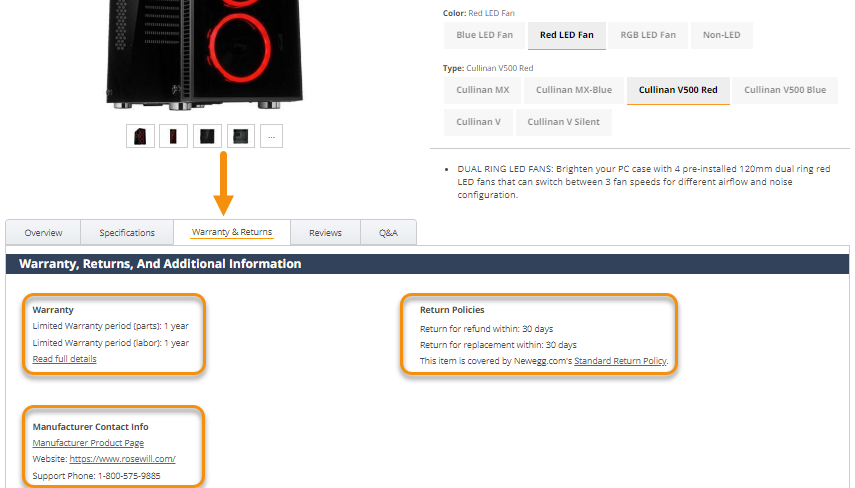This image depicts a company's returns page displayed on a computer screen. Central to the screen is a light gray navigation bar. Just below this bar is a partial view of a sleek black piece of equipment featuring a prominent red LED light ring, likely part of a monitor or a PC case. Directly beneath this main image are five smaller thumbnail images, each offering different perspectives of the equipment.

To the right of the images, text indicates "Color: Red LED Fan," with additional color options available. Below this, the product type is displayed: "Cullion V500 Red," which is highlighted, alongside other model variants.

Beneath the main image and thumbnails, five tabs are arranged horizontally: Overview, Specifications, Warranty and Returns, Reviews, and Q&A. The "Warranty and Returns" tab is currently selected, underlined in gold, and marked with a downward-pointing arrow for emphasis.

Continuing further down, a navy-colored banner prominently reads "Warranty Returns and Additional Information." Below this banner are three rectangular informational bubbles, each with a clear designation: Warranty Information, Manufacturer Contact Info, and Return Policies.